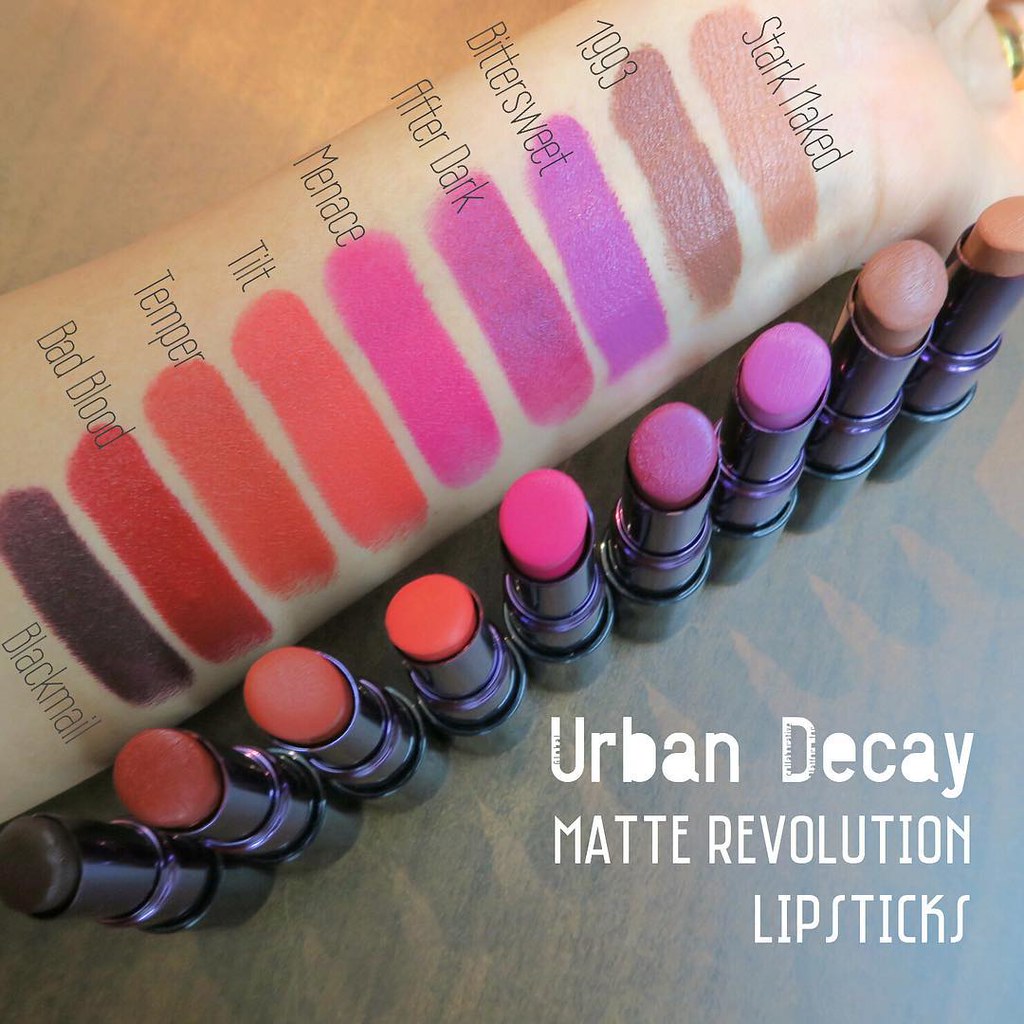The photograph is a detailed makeup advertisement showcasing a variety of Urban Decay Matte Revolution Lipsticks. The scene is set on a brown, wooden table. In the center, an arm is prominently displayed, adorned with multiple lipstick swatches. Each swatch is meticulously labeled with black text, indicating the shade names from bottom left to top right: Blackmail, Bad Blood, Temper, Tilt, Menace, After Dark, Bittersweet, 1993, and Stark Naked. The swatches cover a spectrum from deep reddish-purple to black, pink, brown, purple, and orangish-red. Nearby, the corresponding lipsticks are neatly arranged, reflecting the same color palette. The advertisement is anchored by additional text at the bottom right in white font, which reads "Urban Decay Matte Revolution Lipsticks."